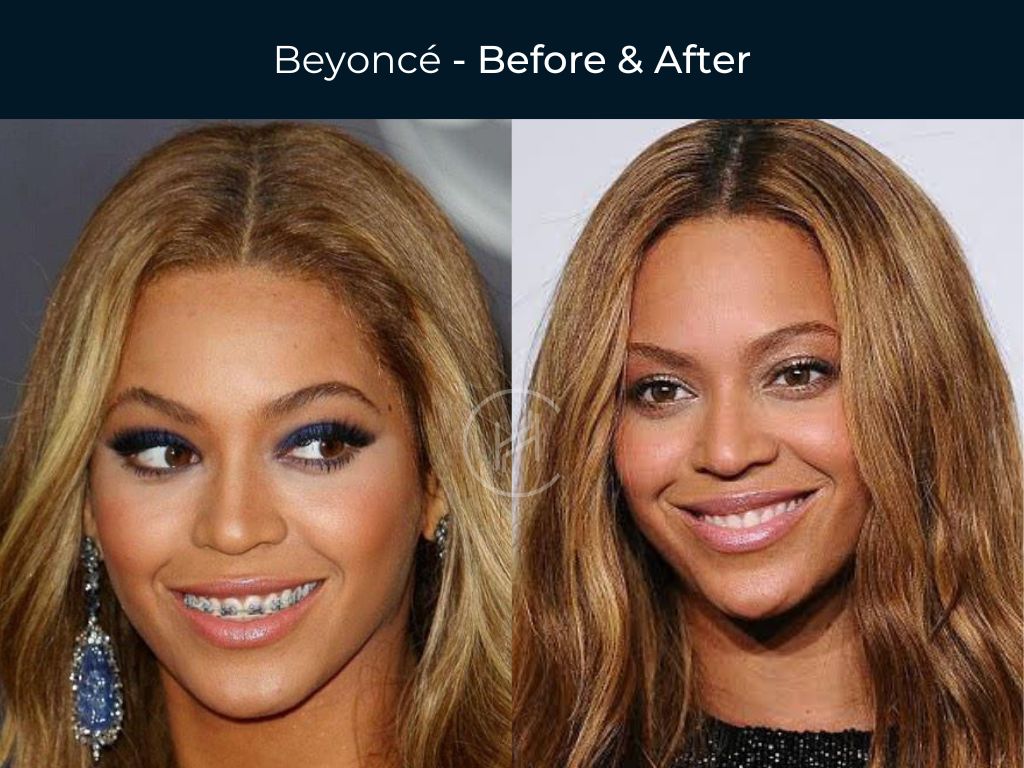The image features a side-by-side comparison of Beyonce, labeled "Beyonce - Before and After." On the left, the younger Beyonce sports a lighter, blondish to light brown hair. Her makeup is more vibrant with blue eyeshadow, mascara, large fake lashes, and bright blue dangly earrings that match the braces on her teeth, displayed in her smile as she looks to her right. The right image, depicting a more contemporary Beyonce, shows her with darker honey blonde hair, which is still long but appears more natural. She is without brases, eyeshadow, or earrings, presenting a more understated makeup look. Despite some subtle age-related changes such as faint wrinkles from frequent smiling, her overall appearance, including her hairstyle and facial features, remains quite similar. Both images focus closely on her face, highlighting her evolving yet consistent beauty over the years.